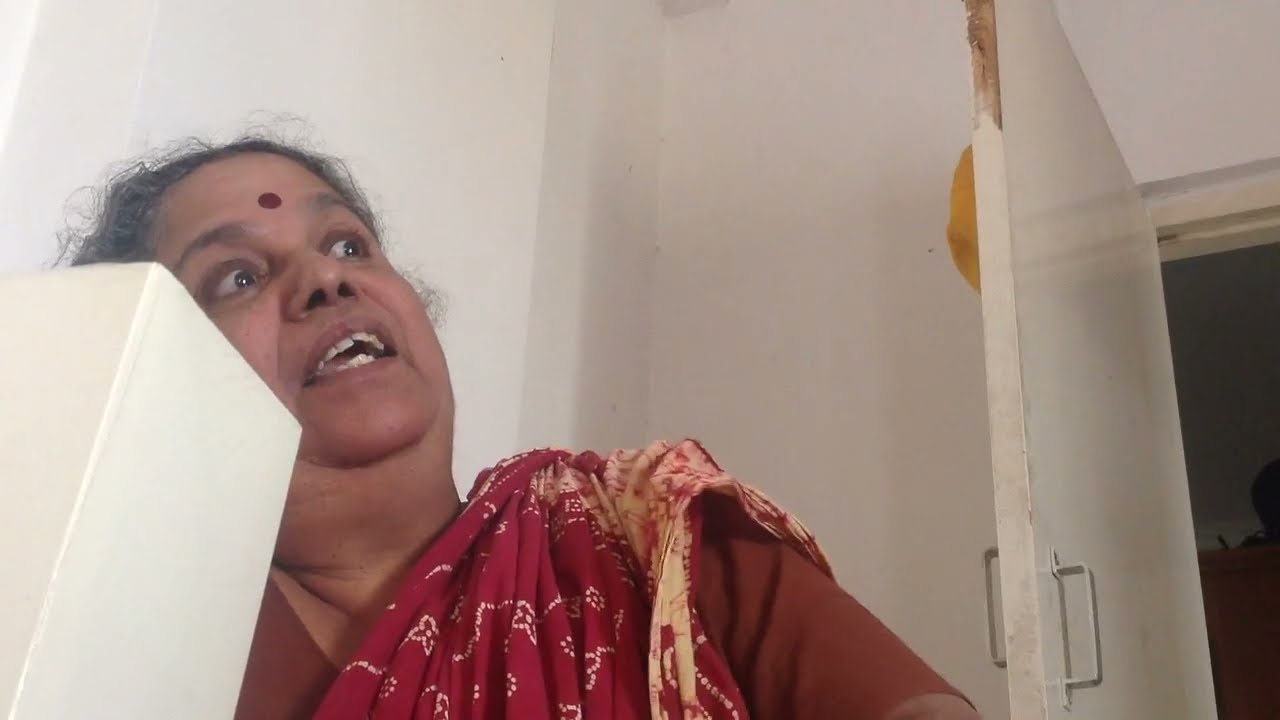This image depicts an indoor scene featuring an Indian woman, characterized by black, slightly wispy hair and a red bindi on her forehead. She appears to be in the midst of talking or singing, with her mouth slightly open and her body leaning at an angle. The woman is adorned in traditional clothing, primarily red with orange and yellow hues and intricate designs. Draped over her shoulders are red coverings, and she wears a gold bracelet on her wrist. Her right arm is raised, with her hand open, although the motion of her hand seems slightly blurred. The background includes white walls, a white pillar next to her, and an open white door to the right side of the image, indicating she is inside a room.